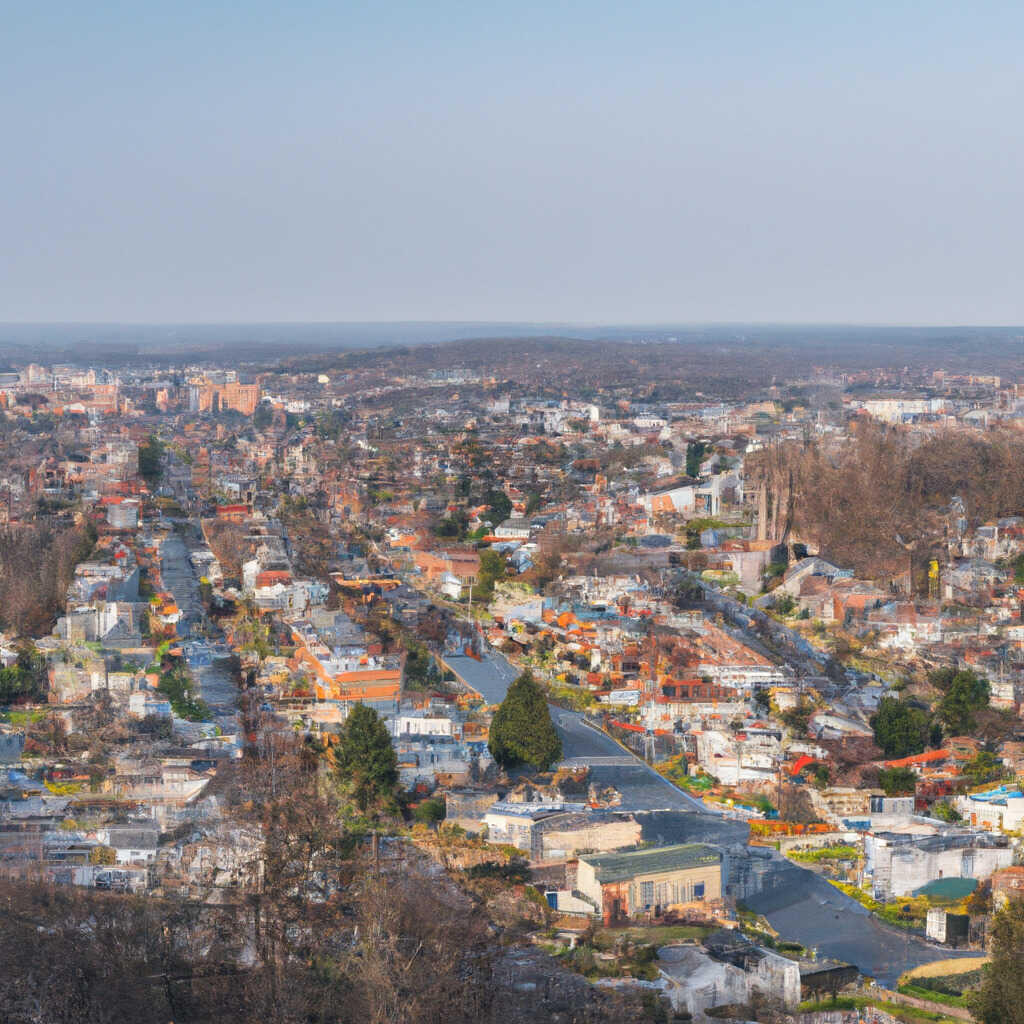This photograph captures an overhead view of a suburban city center during the late afternoon or early evening. The sky is a clear, light blue without any visible clouds, suggesting a calm weather day. The image is divided into thirds, with the top third showing the sky and the bottom two-thirds displaying the cityscape. 

The city below exhibits a mix of residential and possibly some commercial buildings, organized in rows along long paved streets. The buildings vary in color—white, orange, and gray—and have diverse architectural designs and roof shapes. This diversity in design and color adds visual interest to the scene.

Interspersed between the buildings are scattered trees and bushes. Some trees are leafy while others appear to have no branches, suggesting the photograph might have been taken in late summer or early fall. Although vehicles, signs, and power lines are visible, the image is taken from such a height that the finer details of vehicles or people are not discernible.

In the background, there are taller buildings, hinting at a denser part of the city further away from the primarily residential foreground. This elevated perspective provides a broad view of the town, highlighting the extensive spread of homes and the bits of greenery woven into the urban fabric.